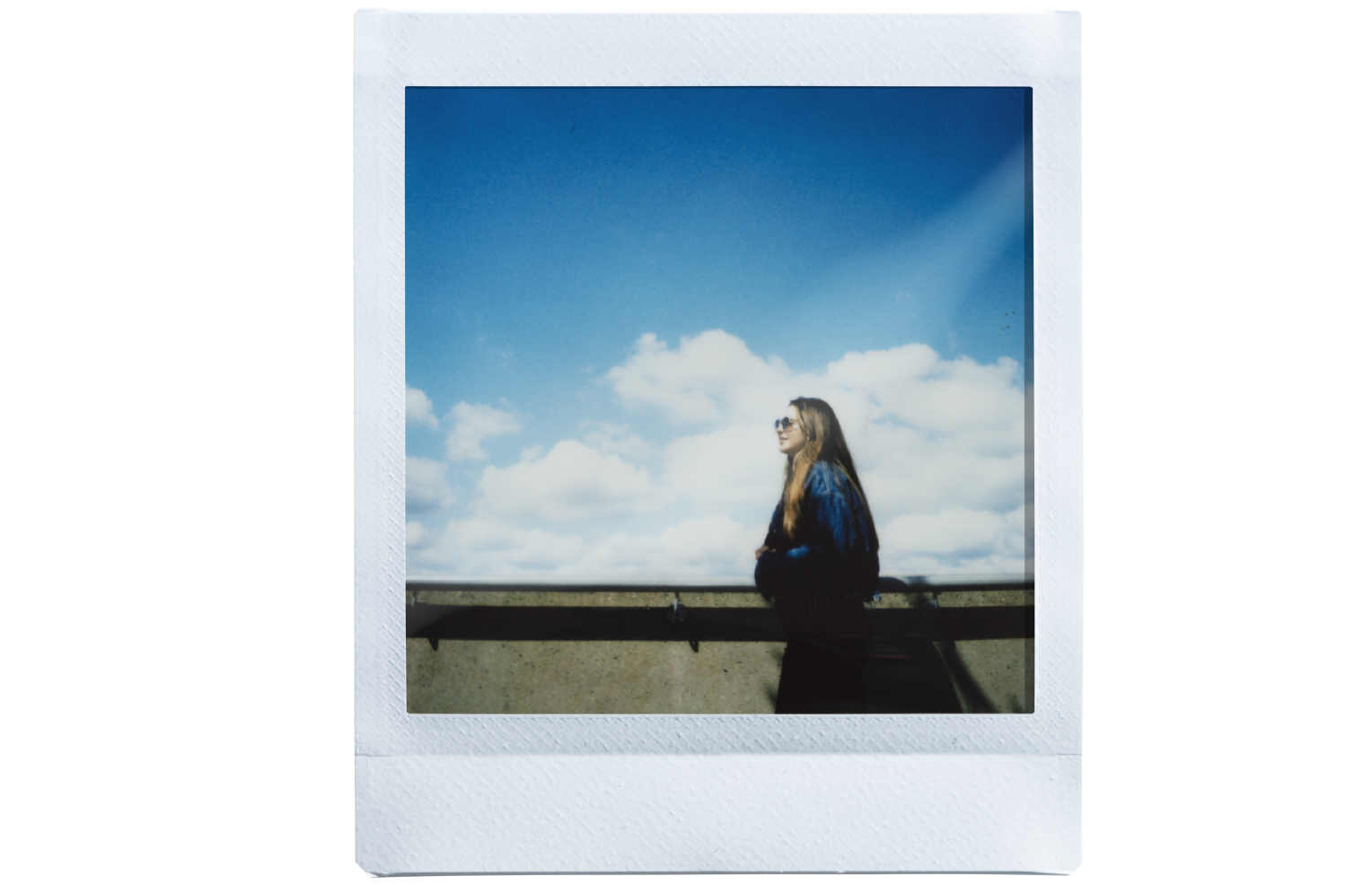In this vintage Polaroid picture, a woman with long, straight brown hair, wearing large sunglasses reminiscent of the 60s or 70s, walks along a wall or banister on a beautiful day. Her attire includes a shiny, possibly silk, jacket or shirt that shimmers in the sunlight, and while her lower half is obscured or not visible, she exudes a sense of carefree movement. The scene captures a sunlit blue sky with fluffy white clouds, enhancing the photograph's nostalgic feel. The image appears to be taken during a bright, sunny day, with detailed shadows hinting at the time of day and the direction of her walk. The Polaroid's characteristic white border adds to its retro aesthetic charm.